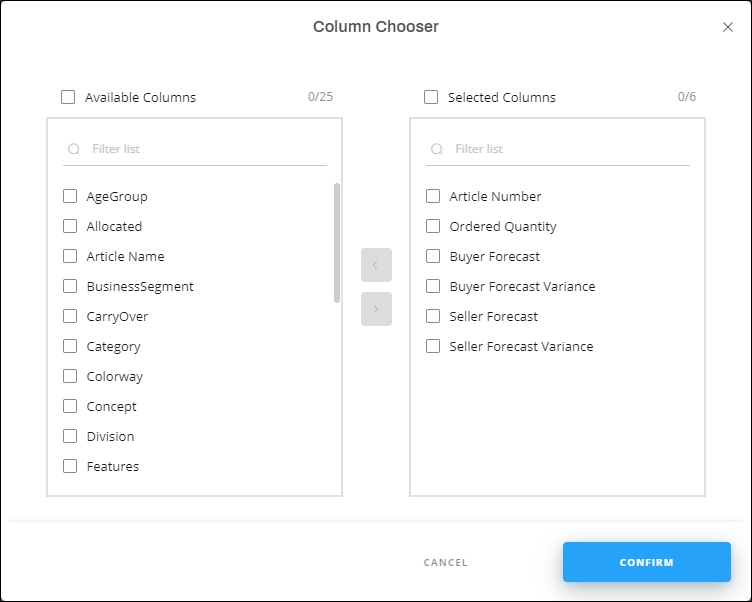The image depicts a detailed interface of a program titled "Spring Trial Bay," which features a column chooser utility. On the left side of the interface, there is a section called "Available Columns" marked with a checkable box labeled as "025." Accompanying this is a search option named "Filter List," enabling users to navigate through the checkable options listed below, which include: age group, allocated article name, business segment, carryover, category, colorway, concept, division, and features.

On the right side, there is another section labeled "Selected Columns 06," displaying items such as article number, order quantity, buyer forecast, buyer forecast variance, seller forecast, and seller forecast variance. Two navigation buttons are positioned in the center, one marked with a ">" for moving items right, and another marked with a "<" for moving items left.

Located at the upper right-hand corner of the interface, an "X" icon provides an option to exit the program. Near the bottom, outside a dividing line, lie two additional buttons: a cancel button on the left and a confirmation button on the right. The confirmation button features white text on a blue background. The overall design sports a predominantly white backdrop with black text, ensuring high readability.